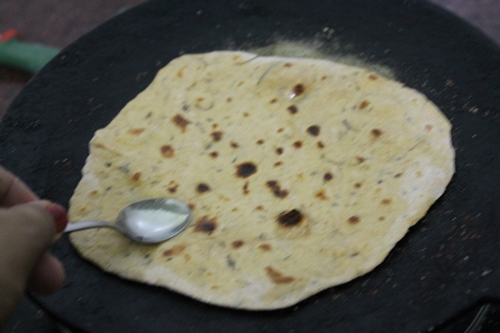In this image, a seemingly large omelet or pancake is shown in a black frying pan. The yolk-colored food item is spread flat and wide, with some black spots and other dark shapes possibly resulting from the cooking process or pan residue. A woman's left hand, adorned with nail polish on her thumb, is visible holding a silver spoon that has sauce on it. She is using the back of the spoon to pat down the pancake-like item to ensure an even spread. In the upper left corner of the image, a green object with a touch of red can be seen, though its exact identity is unclear. The upper part of the food appears lighter, suggesting it may still be cooking. The overall setup indicates a hands-on cooking process in progress, with close attention to detail.